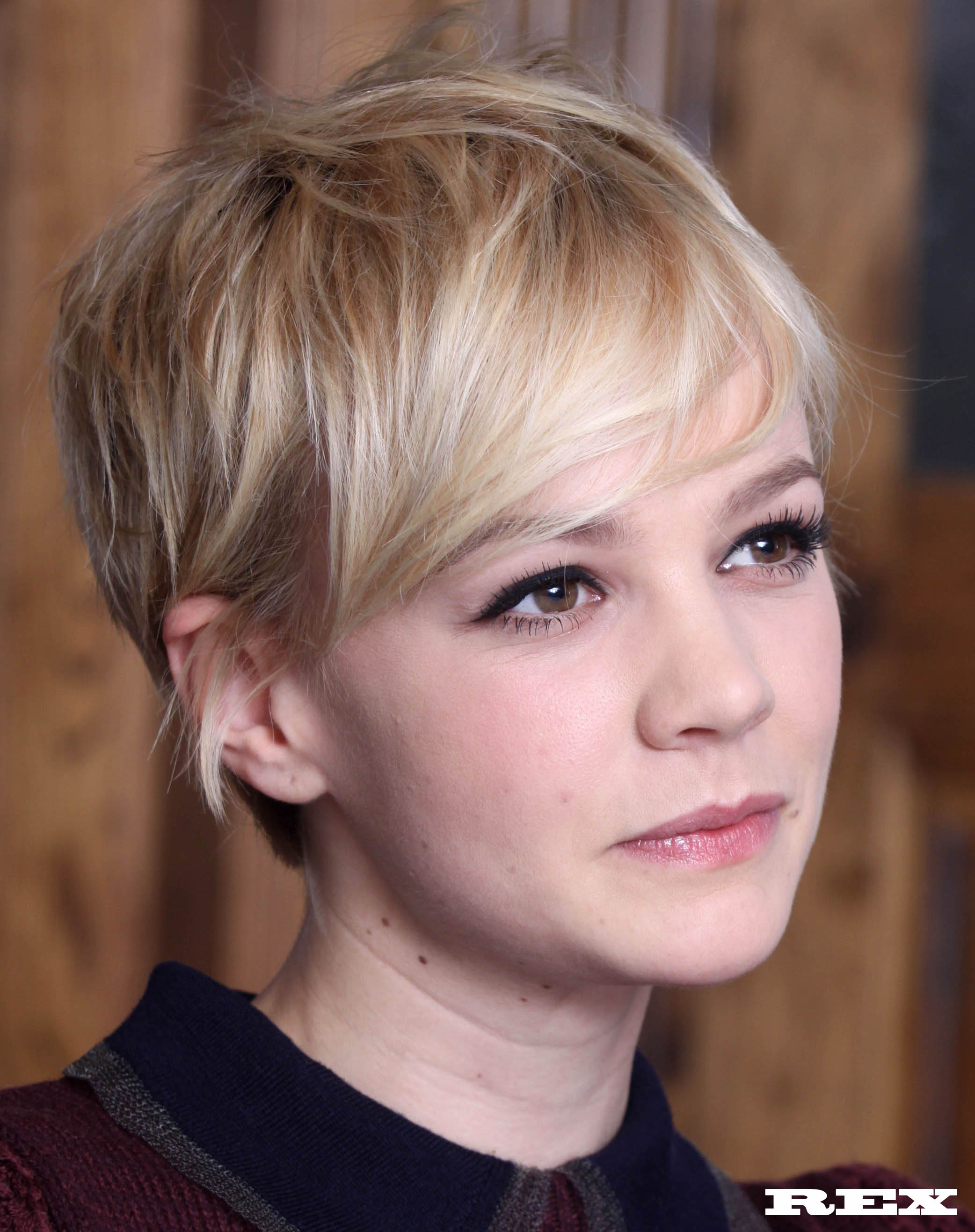The photograph is a professional, promotional shot of an actress with short, wispy, pixie-cut blonde hair styled to the side. She has brown eyes, light makeup accentuated with mascara, and pinkish lipstick. Her attire includes a collared garment visible from just below her neck up; the collar is blue, then gray, transitioning into maroon, with black strings integrated into the top. She gazes dreamily into the distance with a serene, thoughtful expression, giving a faint half-smile. The background is blurred in shades of black and light brown, with no additional people or objects present. The lower right corner of the image features a white watermark text that reads "R-E-X." The lighting and focus are meticulously executed, suggesting the photographer was in close proximity and the actress was aware of being photographed, adding to the image's polished and professional feel.